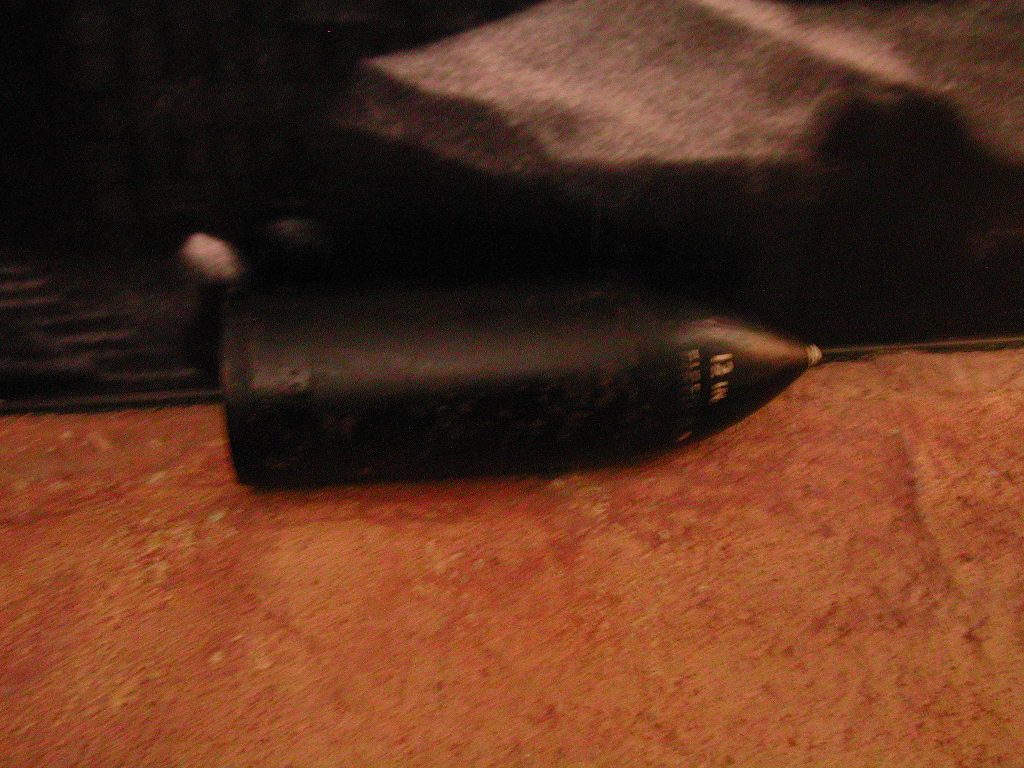The image depicts a black, metallic-looking object resembling a flask or an electronic stirrer, tapered at the top and laying on its side on a reddish-brown stone or carpeted surface. The object's pointed top has a small stem-like protrusion, which may be a stopper or part of the background, and features faint white writing, possibly reading "12IN," though the text is slightly smudged and unclear. The surface behind the object is covered by a large, dark cloth that occupies most of the upper part of the picture, illuminated in some areas by light coming from the mid-right and top middle. The image quality is grainy, and there are indistinguishable white and black objects near the base of the flask.